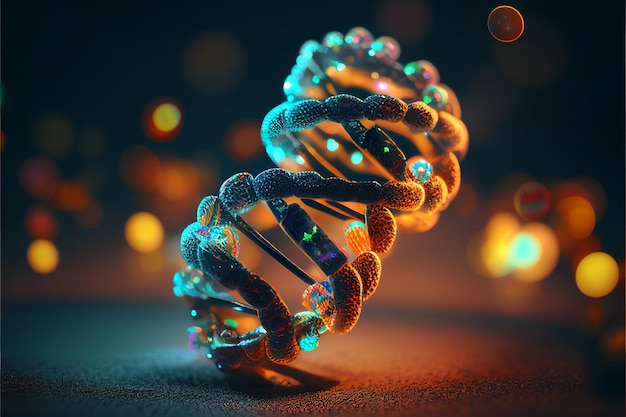The image is a computer-generated graphic of a structure resembling a double helix, likely not DNA but rather an artistic interpretation. The double helix features two strands crisscrossing and spiraling back and forth, adorned with textured oval beads that resemble bumpy little jewels—some iridescent and translucent. The helix appears anti-gravitationally tilted, giving the impression that it is both falling and perfectly upright. It rests on a soft matte surface with warm golden and amber lights in the blurred background, exhibiting a bokeh effect. Additionally, there is a small, solid circle or button-like object at the top right, and a cool light blue illumination from the left, adding a variety of colors such as blue, yellow, and red to the scene. The backdrop is predominantly warm tones with a mixture of flare lights, giving the whole image a magical, glowing ambiance.